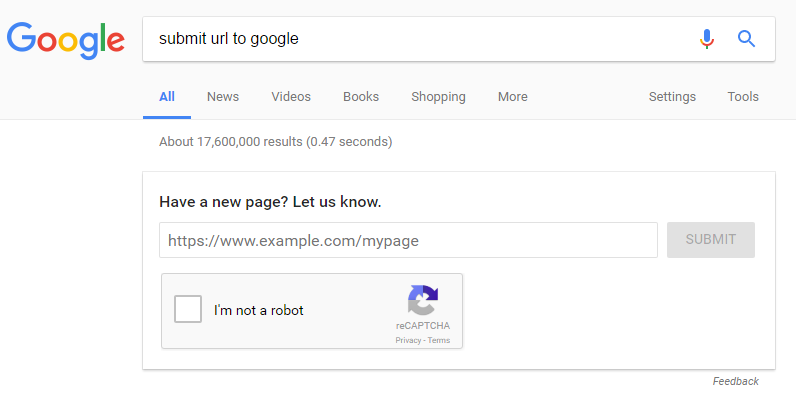The screenshot depicts a partial view of a website, emulating what appears to be a Google Search results page. At the top left corner, the colorful "Google" logo is prominently displayed. Below the logo, a search bar contains the query "submit URL to Google." To the right of the search bar, icons for a microphone and a magnifying glass (indicating voice search and search action respectively) are visible. Beneath the search bar, navigation tabs labelled "All," "News," "Videos," "Books," "Shopping," "More," "Settings," and "Tools" are arranged horizontally.

Just below these navigation tabs, the text "About 17,600,000 results (0.47 seconds)" indicates the number of search results and the speed of the search. Following this, a prominent section highlights an action box with the heading "Have a new page? Let us know." Inside this box, there is a text field pre-filled with the URL "https://www.example.com.mypage." To the right of this field, a blue "Submit" button is positioned. Below this, a CAPTCHA verification section is presented, featuring a checkbox accompanied by the text "I'm not a robot" alongside a CAPTCHA logo, signaling a security measure to ensure a human user interaction. The overall design and layout closely mimic the familiar interface of Google’s search result page.